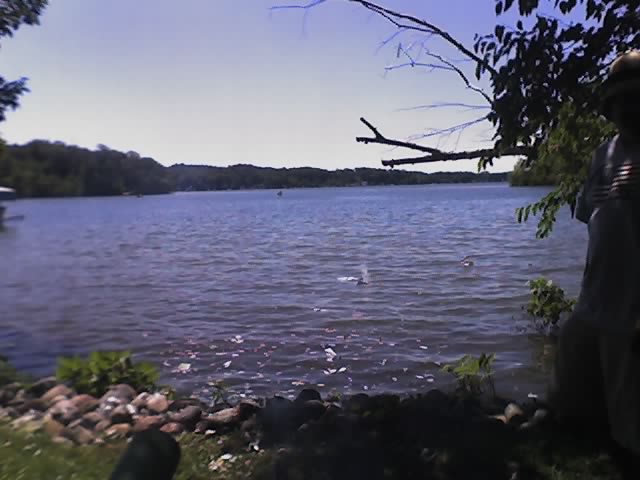The photograph depicts a serene lakeside scene, framed within a rectangular, horizontally-oriented composition. In the foreground, the shoreline is detailed with grass and an array of stones, adding texture to the scene. On the right side, partially shadowed, stands a figure whose gender is indistinct, potentially a woman, beside a tree that extends its branches and leaves into the upper right of the image. The lake itself, deep blue in color and devoid of boats, stretches across the center of the photograph, bordered in the distance by a land strip of trees and hills extending from left to right. The sky, occupying the top third of the image, transitions from a clear light blue at the horizon to a deeper blue, highlighting the tranquil, almost autumnal atmosphere of the scene.